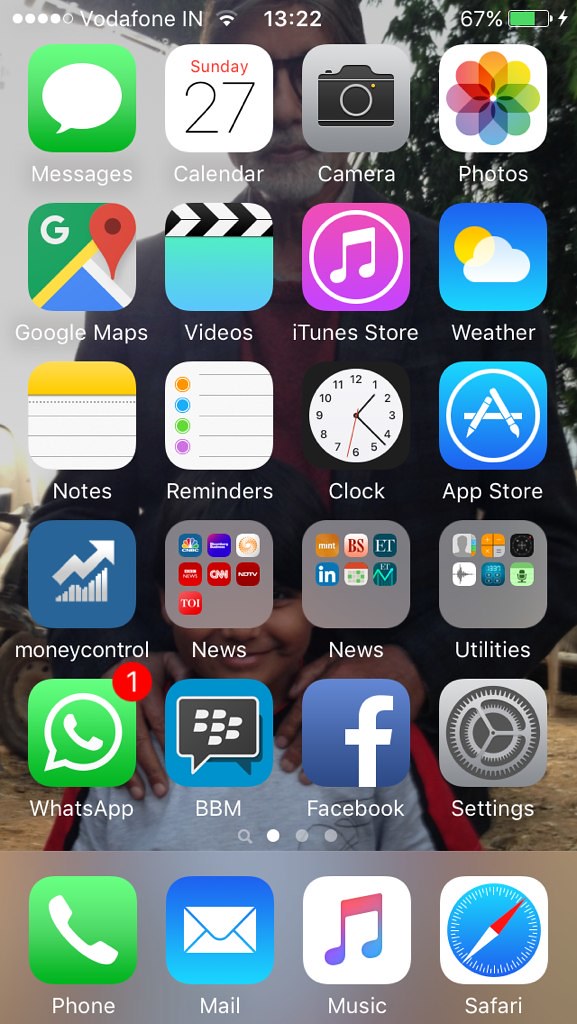The image is a screenshot of an iPhone screen with a heartfelt background photo of an older gentleman wearing glasses and a young boy with dark hair and bangs. Both are facing the camera; the boy is smiling brightly, while the gentleman offers a gentle, slight smile, resting his hands on the boy's shoulders. The boy is clad in a long-sleeved gray, black, and red shirt.

The iPhone screen is populated with a variety of app icons arranged in rows. The first row features Messages, Calendar, Camera, and Photos. The next row includes Google Maps, Videos, iTunes Store, and Weather. Following that, the third row comprises Notes, Reminders, Clock, and App Store. The fourth row includes two apps, Money and Control, accompanied by three grouped folders labeled ‘News’, ‘News and Utilities’, and another folder also named ‘News’. The fifth row displays icons for WhatsApp, BBM, Facebook, and Settings.

At the bottom of the screen, the dock holds the Phone, Mail, Music, and Safari icons. The status bar at the top shows the current time as 13:22, the carrier as Vodafone IN, a Wi-Fi symbol with two bars, and a battery level at 67%. 

This detailed visual depiction of the iPhone screen reflects a mix of personal warmth and everyday digital functionality.